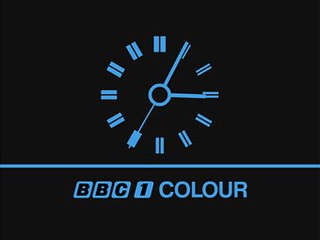This image showcases a computer-generated logo set against a solid black background. Centrally positioned is a clock displaying the time 3:05, with the second hand precisely on the 7. The clock's face features Roman numerals for the hour markers and lacks a surrounding frame, giving it a minimalist appearance. Beneath the clock, a light blue horizontal line spans from the left to the right of the image, providing a visual anchor. Directly below this line, the text "BBC1 Color" is prominently displayed. The letters "BBC1" appear as stylized keyboard keys, featuring black writing on a blue background, while the word "Color" is rendered in a matching blue font. The overall design is sleek, modern, and visually striking.